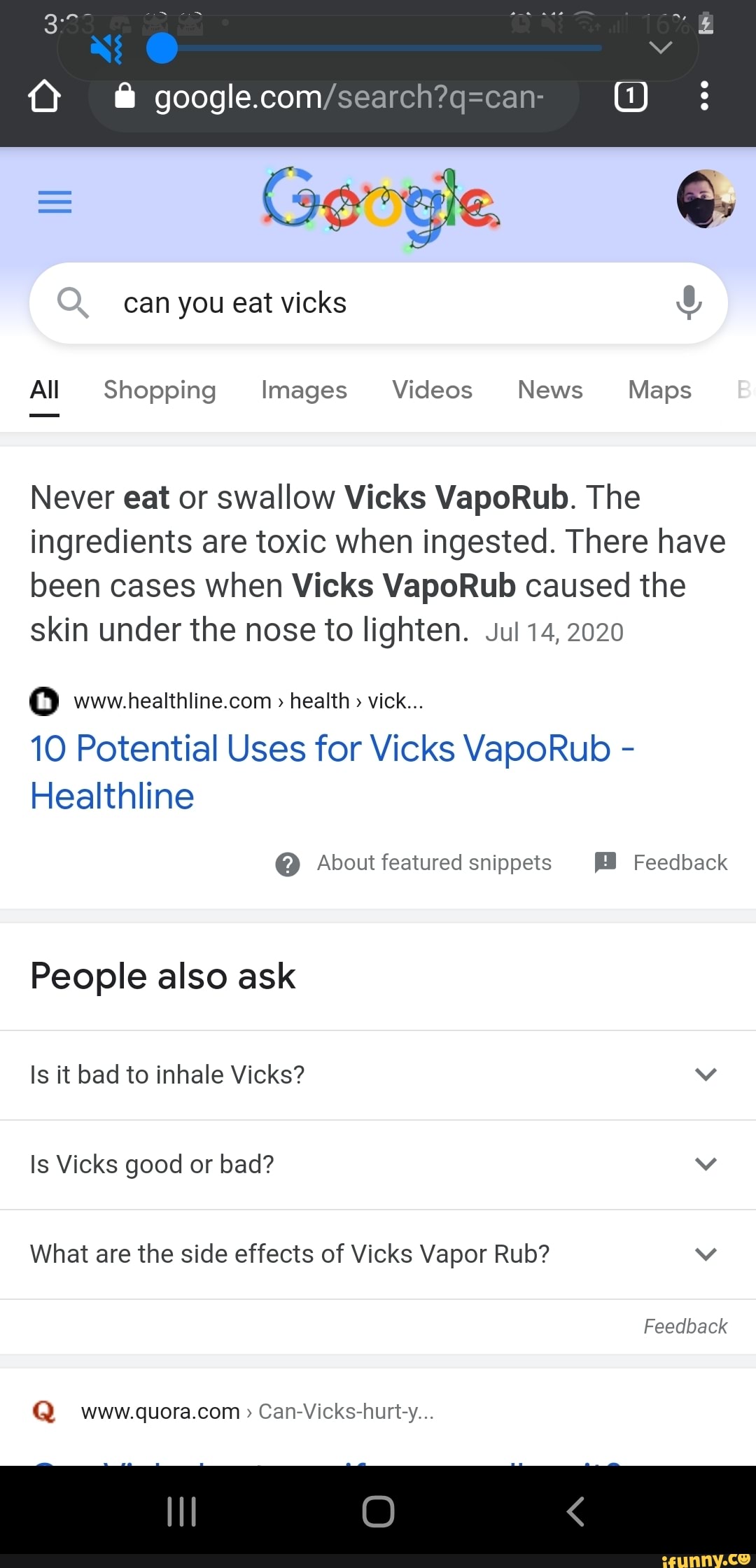This image is a screenshot from a Google search on an Android device in dark mode. The bottom part of the screen displays the navigation buttons on a black bar, while the top shows the volume control slider, which is set all the way to the left, indicating that the device is muted. The symbols at the top also include a speaker icon with a slash through it, representing the muted state.

The Google search query typed in is "can you eat Vicks," referring to Vicks VapoRub. The search results clearly state, "Never eat or swallow Vicks VapoRub. The ingredients are toxic when ingested," followed by a cautionary note about the product causing skin lightening under the nose in some cases.

The header of the Google homepage features festive Christmas lights around the Google logo, suggesting that the search was conducted during the holiday season. Additionally, at the bottom of the screenshot, there appears to be a yellow watermark that reads "ifunny.co", indicating the source or platform where the screenshot might have been shared.